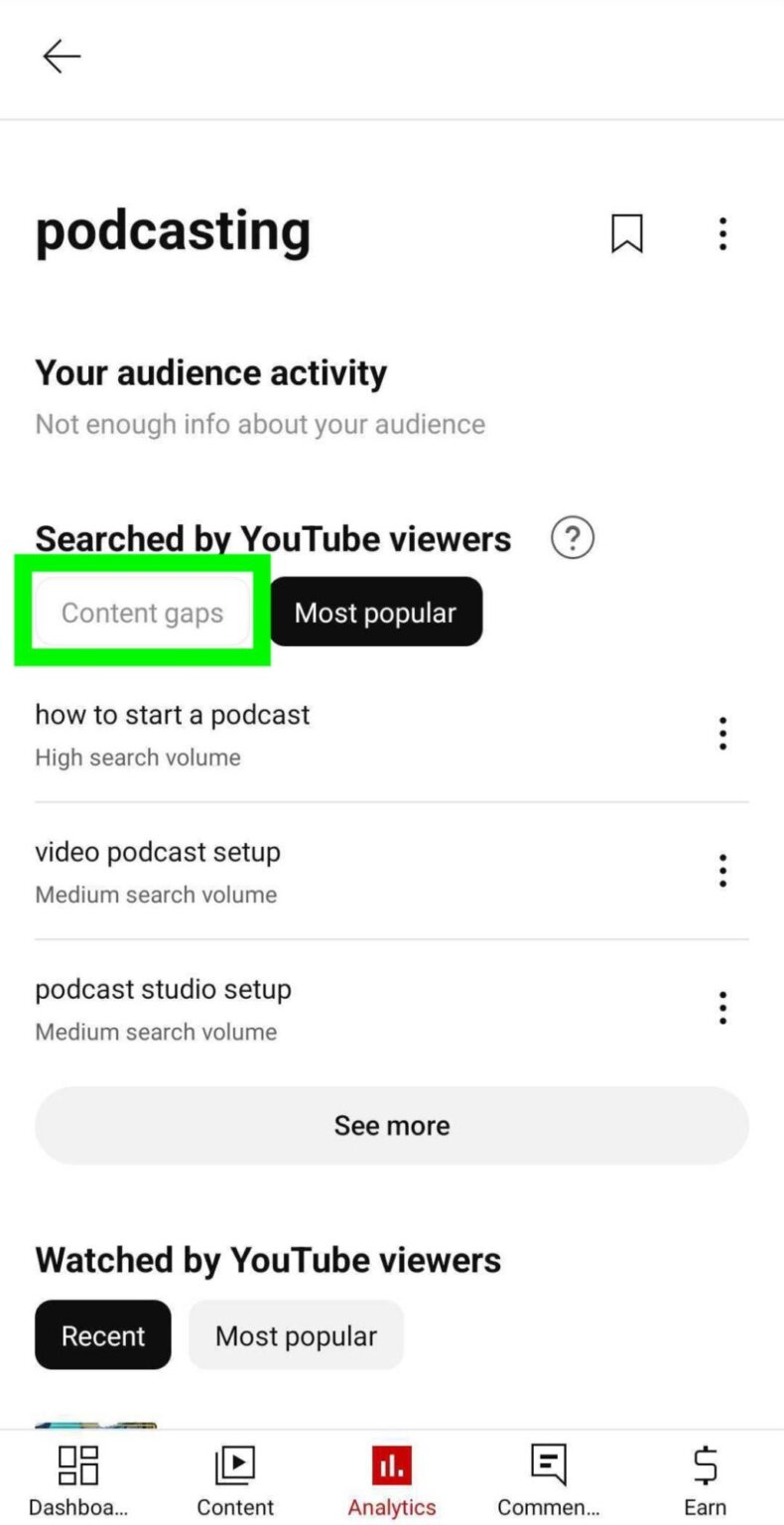The image is a screenshot taken from a mobile device. At the top left corner, there is an arrow pointing to the left, indicating a back navigation option. The screen has a white background with a thin gray horizontal bar running across the top. Below this bar, in bold black text, it reads "Podcasting." Underneath, there is another line of black text stating "Your audience activity," followed by a gray subtext that reads "Not enough info about your audience."

On the top right, three vertical dots are visible, indicating a menu or additional options. Below these elements, there is a unique shape resembling a square with the bottom pushed up into a triangle. Directly under this shape, the text "Search by YouTube viewers" is displayed along with a small question mark icon enclosed in a circle.

Further down, the section titled "Content Gaps" is highlighted with a green rectangle. Following this, there is a black button with white text that says "Most popular." Below this, a list of search terms is shown:

1. "How to start a podcast" - tagged as high search volume.
2. "Video podcast setup" - tagged as medium search volume.
3. "Podcast studio setup" - also tagged as medium search volume.

At the bottom of the list, there is a gray button labeled "See more." The phrase "Watched by YouTube viewers" is displayed at the very bottom, followed by two buttons: a black one labeled "Recent" and a gray one labeled "Most popular."